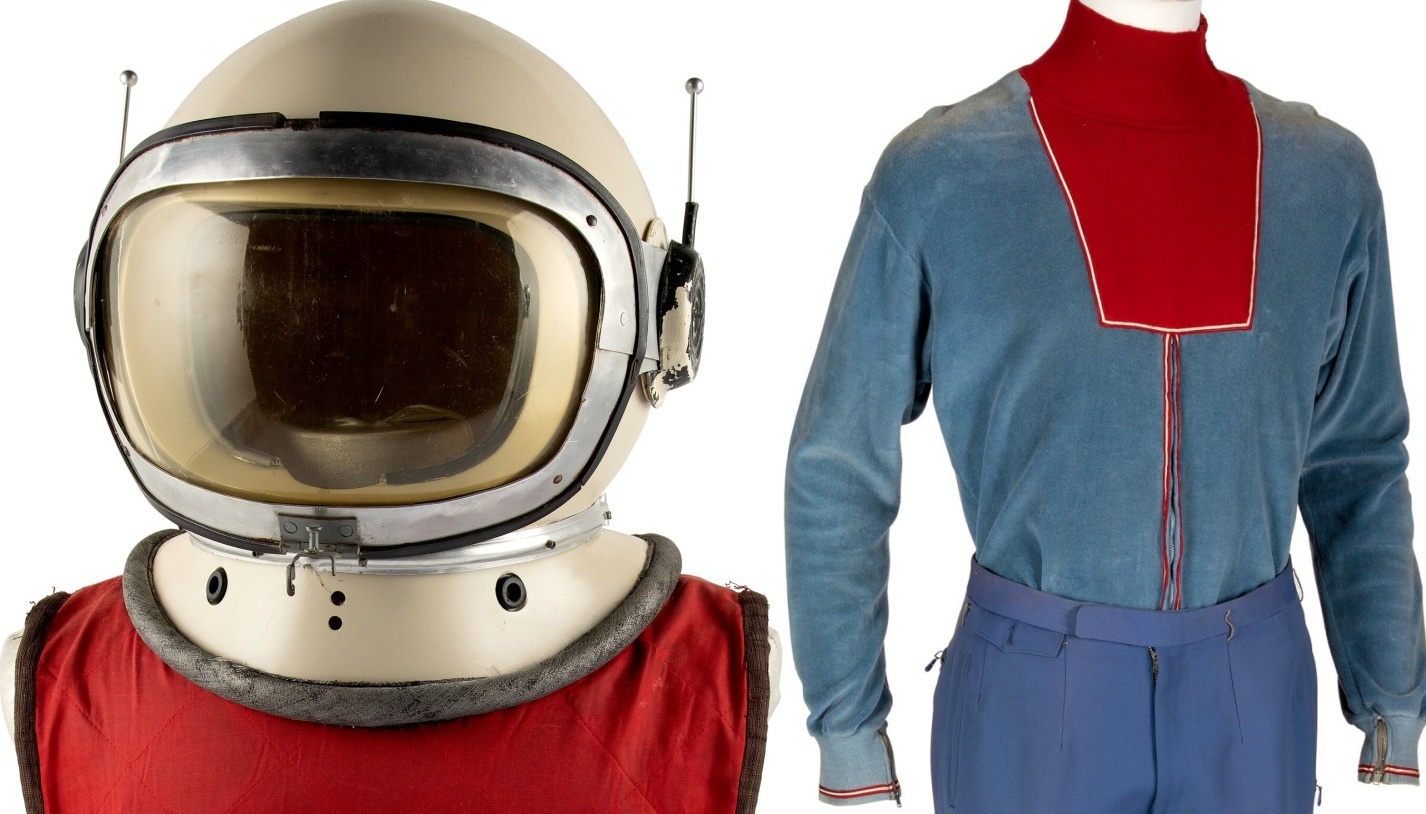The image is a landscape-oriented photograph divided into two sections. The left side of the image prominently features a vintage-style space helmet that covers the entire head. This helmet is round, with a pearly off-white, cream-colored surface, and is equipped with a pair of small antennas on either side where the ears would be. The helmet's neck area is wide and padded in gray with a red bib or collar underneath, and the front has a large, clear visor bordered by stainless steel, silver material. On the right side of the image, the mannequin displaying the rest of the cosmonaut suit is visible. The suit consists of a top with a red turtleneck extending down to the chest and a light blue velvet shirt with red trim. The lower part showcases regular dark blue nylon pants, contrasting with the unique design of the top. Overall, the suit exhibits a distinct East European vibe, enhancing its sci-fi aesthetic.